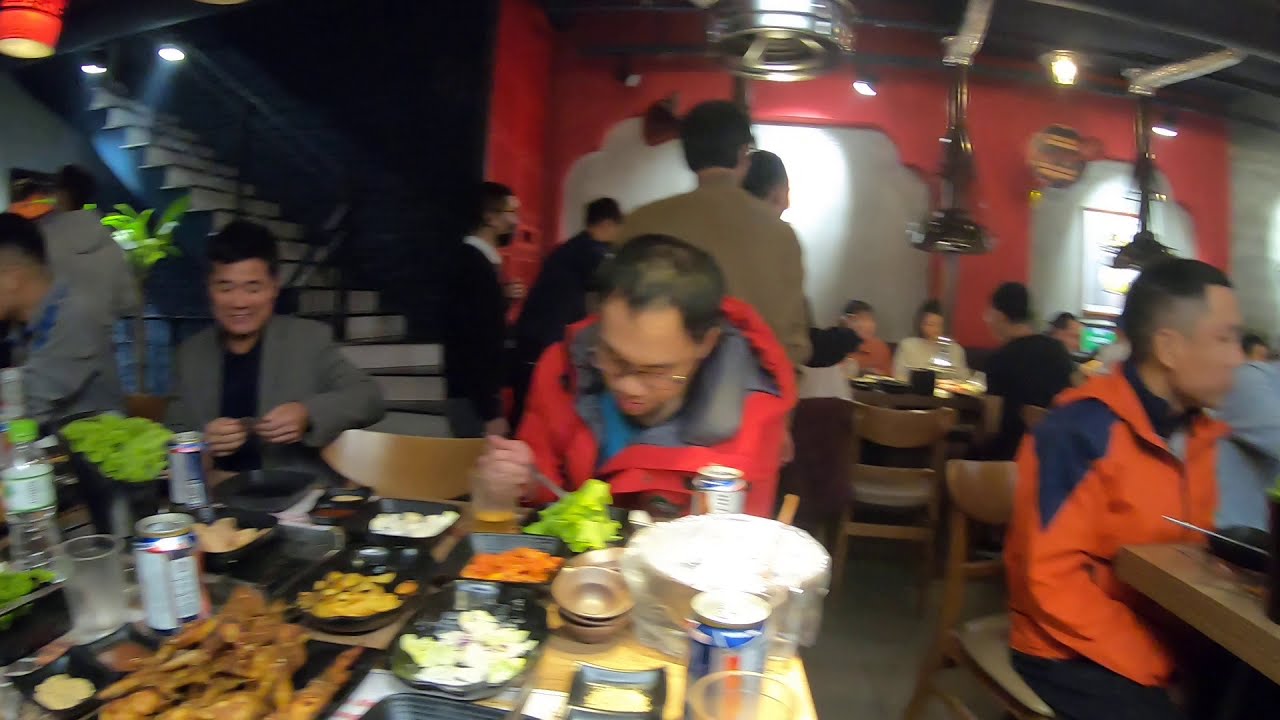The image depicts a bustling dining hall or restaurant setting featuring several occupied tables, primarily with Asian individuals. The foreground highlights three main figures in varying attire. To the left, a man in a gray suit with a black shirt is seen holding something in both hands, smiling downwards with eyes partially closed. In the center, a man in a distinctive red jacket, short hair, and glasses is eating green leafy food from a black plate using a fork. To the right, a man in an orange jacket adorned with blue triangles on the shoulders is seated, looking away to the side. All the tables are laden with a variety of foods, including deep-fried items resembling chicken fingers, orange-colored dishes, possibly akin to macaroni and cheese, and numerous bowls of greens, salads, and carrot slices. Various black containers and several blue, white-labeled cans, likely beers, are scattered across the tables. The setting is framed by a red wall adorned with silver cylindrical pendant lights from the ceiling, and a white staircase leading upwards, part of which is juxtaposed against a dark green-blue wall in the background. The scene captures a lively atmosphere with people both sitting and standing in interactions.